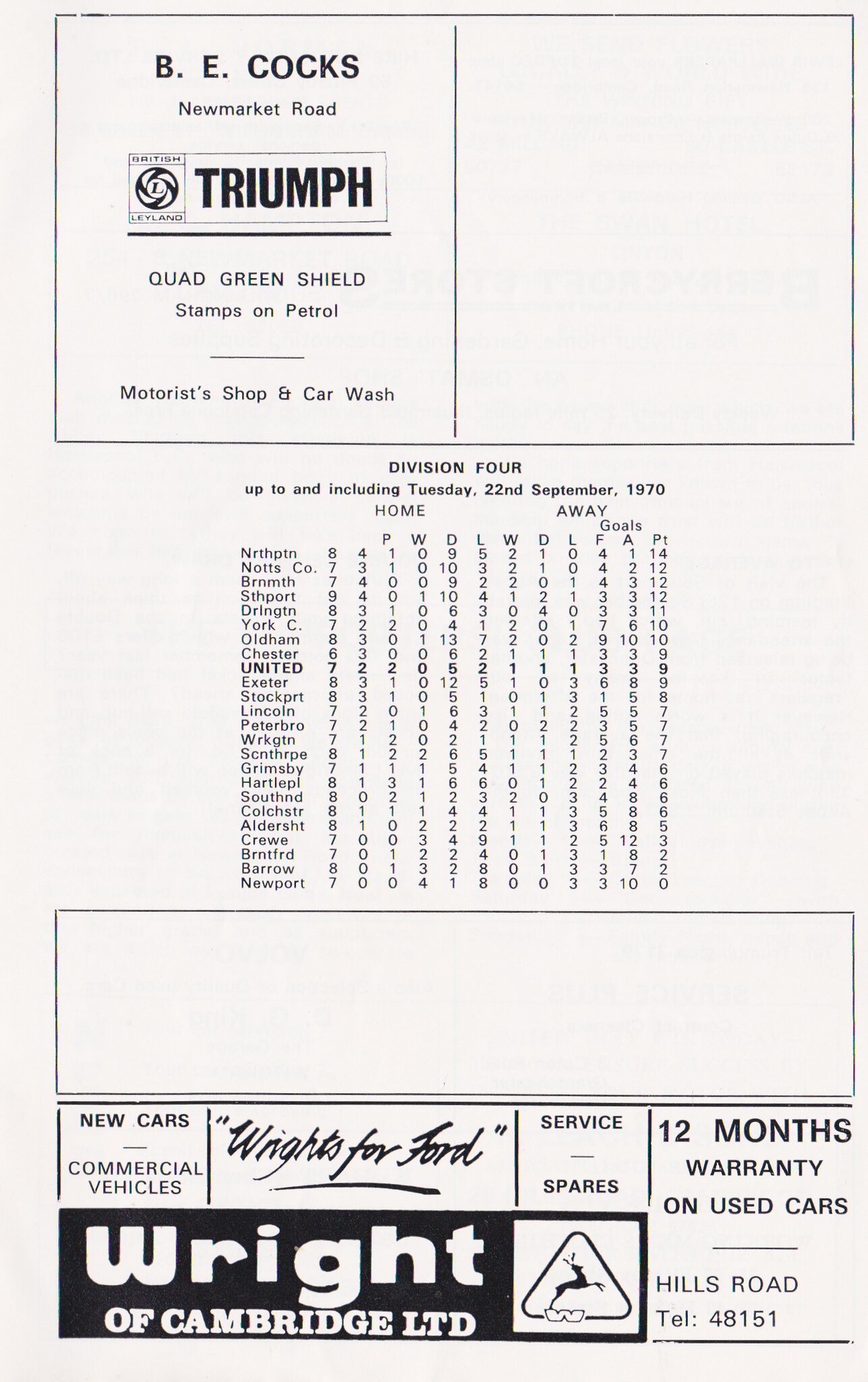This detailed black and white image, likely scanned from a sports program booklet, documents Division IV European soccer team statistics up until Tuesday, September 22, 1970. The page is taller than it is wide and has a slightly off-colored, yellowish-gray background. 

At the top left, there’s an advertisement in bold print for B.E. Cox, New Market Road, featuring services such as Triumph, Quad Green Shield Stamps on Petrol, Motorist Shop, and Car Wash. The top right contains a blank square where an ad could be placed. Centered below, the heading "Division 4 up to and including Tuesday, 22nd September 1970" precedes a grid tracking each team's performance with columns labeled P (Played), W (Won), D (Drawn), L (Lost), F (Goals For), and A (Goals Against).

Beneath the grid, a blank horizontal rectangle awaits another advertisement. The lower section of the page is filled with ads, including a prominent one for a car dealership, "New Cars, Commercial Vehicles, Rights for Ford, Rights of Cambridge LTD," offering service, spares, 12 months warranty on used cars, located on Hills Road with the telephone number 48151. The entire composition suggests this is an archival page, capturing a historical snapshot of soccer standings and local commerce of that time.